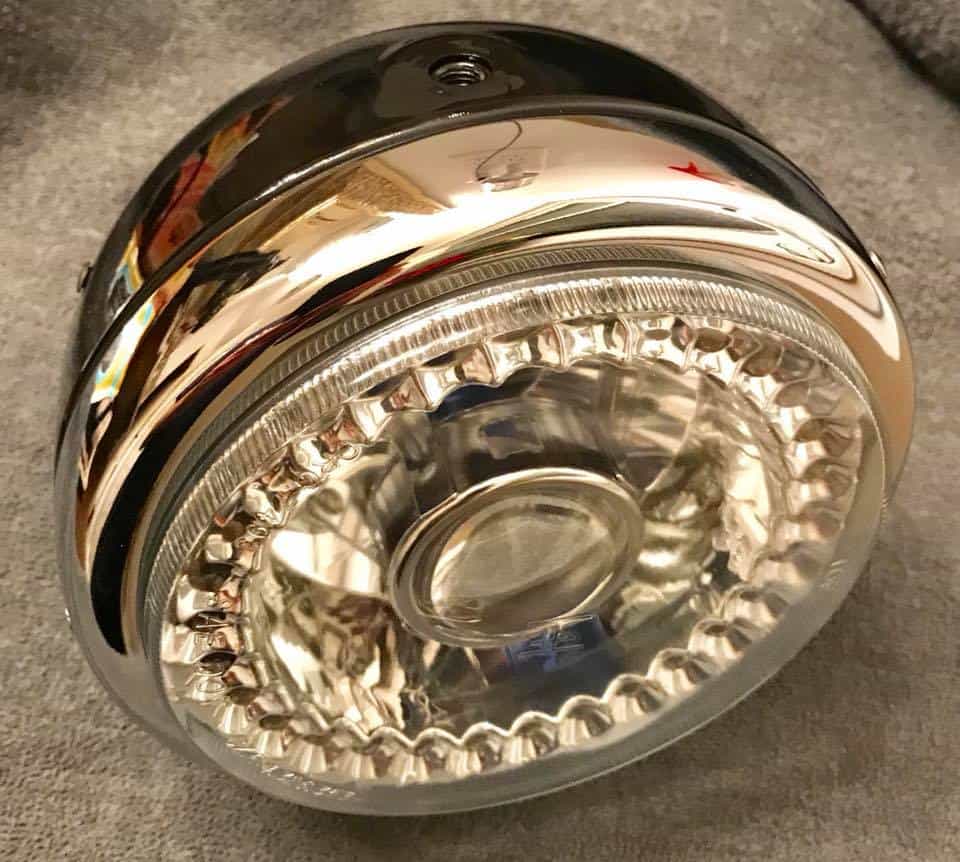The image depicts a close-up view of a metal, circular object that bears a strong resemblance to a light fixture. It features a lid with a glass front, which has ridges along its edges, and a central circular disc that appears functional, perhaps for unscrewing or adjusting the lid. The object also has a silverish section that is bowl-shaped and might be part of its casing. The back of the object includes a hole, suggesting it can be mounted or screwed into place. The item rests on a tan, carpeted or velvety surface, likely in an indoor setting such as a living room. The colors of the object range from silver to a darker shade, possibly gray or black, in the back portion, giving it a polished and somewhat sophisticated appearance.